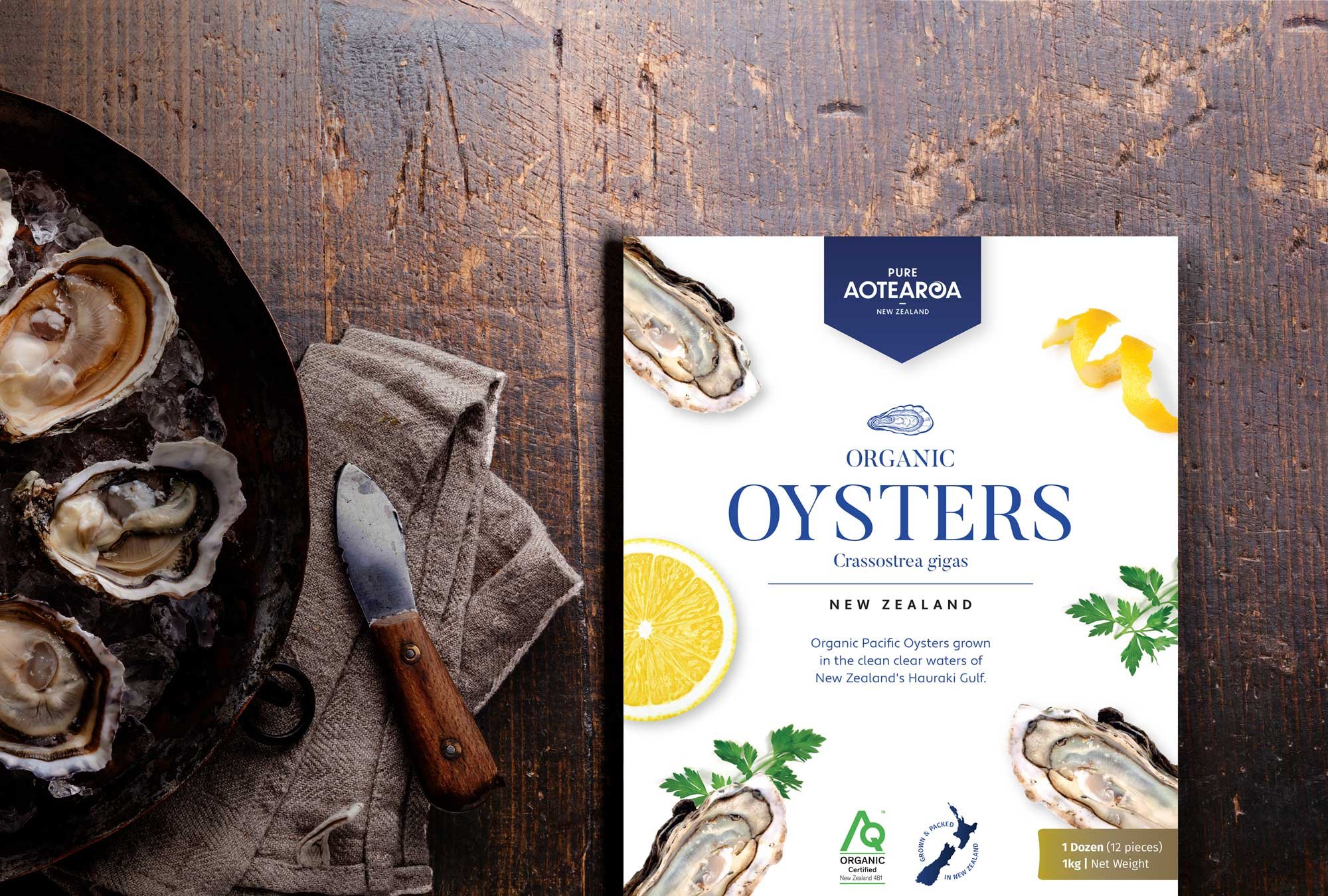On a rustic, well-worn solid oak table adorned with various cut marks and dents, a scene is meticulously set. On the left-hand side, a pan filled with freshly shucked oysters sits invitingly. Next to the pan lies a small knife, presumably used for wedging open the oysters; its wooden handle, secured by rivets, shows signs of frequent use. A cloth for wiping the knife rests nearby. To the right of this setup is a predominantly white book, its cover adorned with enticing images of oysters, lemon slices, and perhaps mint leaves. The book prominently features the title "Organic Oysters" in large font, with the words "New Zealand organic Pacific oysters grown in the clean, clear waters of New Zealand's Hauraki Gulf" detailed underneath. "Oysters" is particularly emphasized on the cover, with "organic" and "New Zealand" in progressively smaller fonts but no less significant in their own right. This book seems to be a dedicated guide to the organic oysters of New Zealand, promising a deep dive into the subject matter.